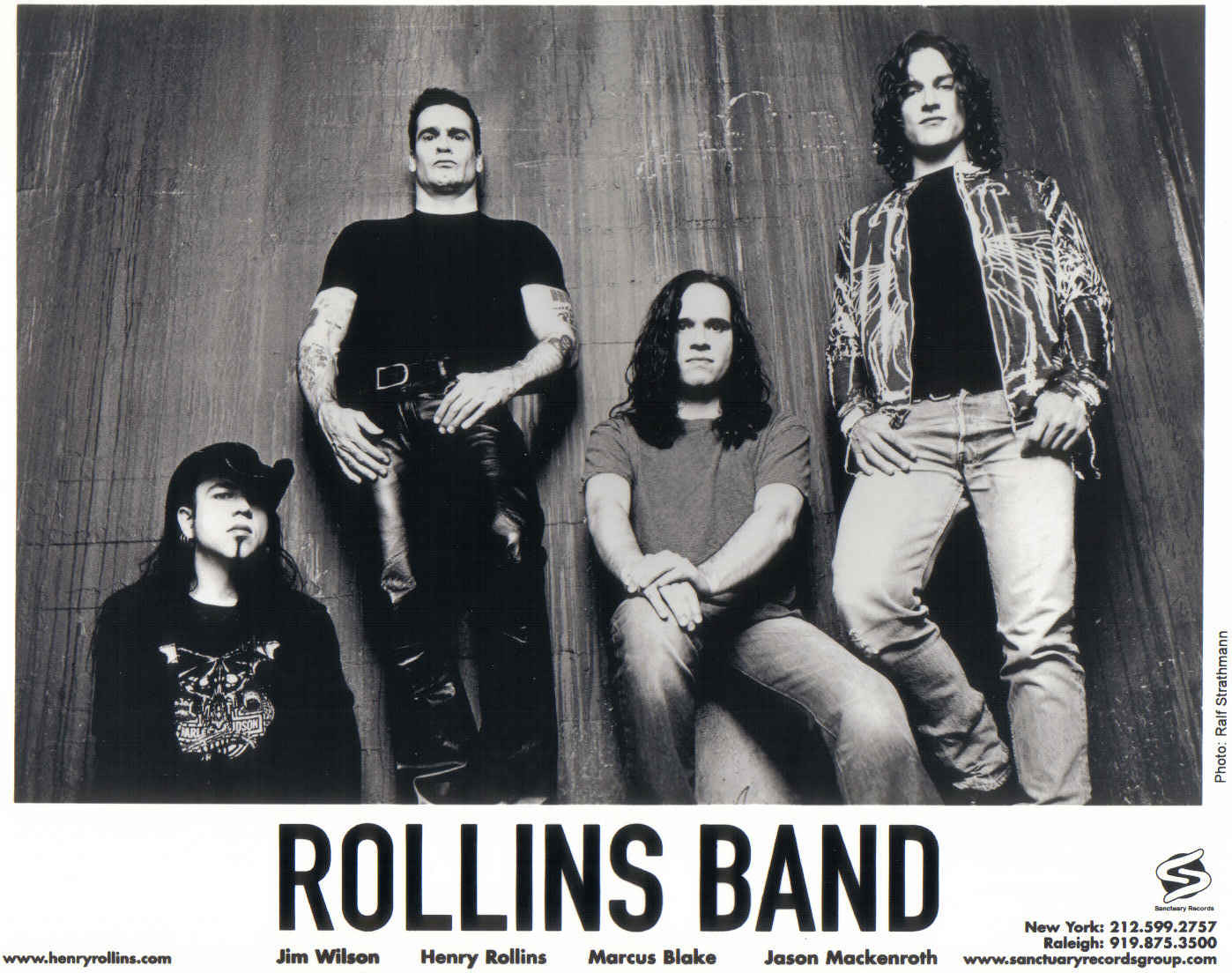In this black-and-white promotional image for the Rollins Band, four members are centered against a concrete wall with dark streaks, creating a gritty, urban backdrop. From left to right, the lineup features: 

- Jim Wilson, who is kneeling and sporting a cowboy hat, a distinctive beard, a shirt with a symbol, and dark attire.
- Henry Rollins, standing upright in a black t-shirt and leather pants, covered with tattoos, exuding a serious demeanor.
- Marcus Blake, seated with long shoulder-length hair, wearing a t-shirt and jeans, with his hands resting one on top of the other, also with a serious expression.
- Jason McEnroth, standing in jeans, a black t-shirt, and a tie-dyed over shirt, his long, curly hair adding to the rock aesthetic.

The text beneath the image prominently displays "Rollins Band," followed by the band members' names: Jim Wilson, Henry Rollins, Marcus Blake, and Jason McEnroth. Additional information includes the website www.henryrollins.com, the record label www.sanctuaryrecordsgroups.com, and mentions of New York and Raleigh locations, alongside their phone numbers. The logo in the bottom right corner features two snakes. The photo is credited to Ralph Stratham.